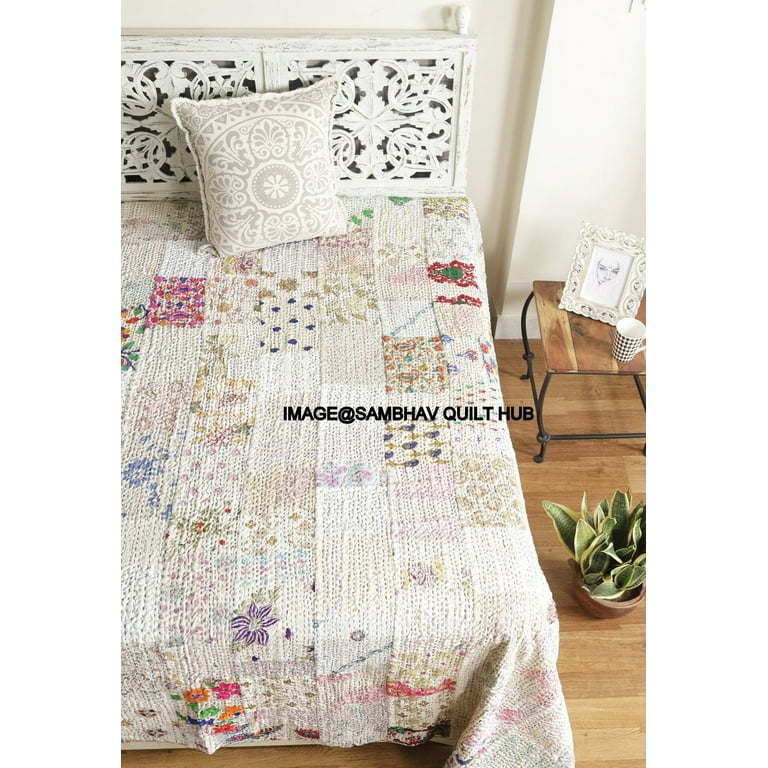This photograph captures a tranquil bedroom scene from an elevated angle. Dominating the image is a cozy bed adorned with a patchwork quilt featuring soothing pastel shades of off-white, tan, blue, and pink squares, some with floral or paisley designs. The bed, framed in ornate white wood, includes a decorative gray and white pillow positioned at an angle. A watermark at the center of the image reads "IMAGE AT SAMBHAV QUILT HUB" in all caps, subtly layered over the quilt. Adjacent to the bed is an end table with a brown wooden top and metal legs, holding a framed drawing and a coffee cup with a checkered pattern. A vibrant green plant in a terracotta pot adds a touch of nature, resting on the wooden plank flooring beside the bed.